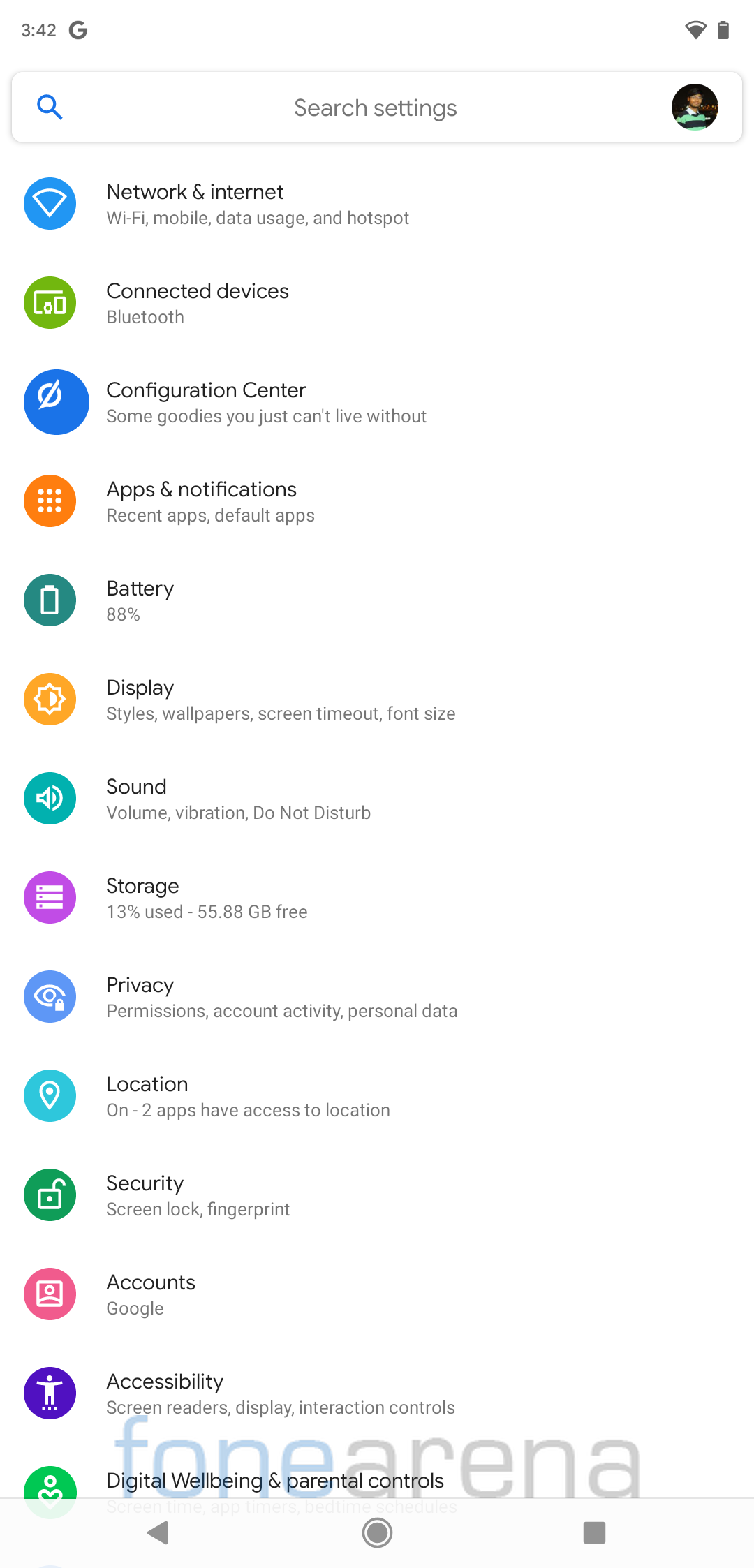Screenshot of a smartphone settings menu displayed at 3:42 PM. The top right corner shows the Google icon, indicating an unread message from Google, Wi-Fi connection, and a nearly full battery. The search settings context menu is at the top. The settings icons from top to bottom are:

1. **Network & Internet** - Depicted by a football diamond with a blue background.
2. **Connected Devices** - Green circle with blue squares.
3. **Apps & Notifications** - Blue circle with a white crossed-out circle.
4. **Battery** - Orange circle with multiple dots.
5. **Display** - Dark green background, icon showing a sun split into half dark and half light.
6. **Sound** - Speaker emitting sound waves.
7. **Storage** - Three rectangles with dots on them.
8. **Privacy** - An eye with a lock at the bottom right.
9. **Location** - A blue icon with a downward pointer.
10. **Security** - Green background with a white unlocked lock icon.
11. **Accounts** - White portrait in a pink circle.
12. **Accessibility** - Figure with arms outstretched, purple background with three dots at the bottom.
13. **Digital Wellbeing & Parental Controls** - Icon not specified in speech, likely relevant to context menu options.

The background of the settings menu is white with black text and the icons on the left-hand side for each option.